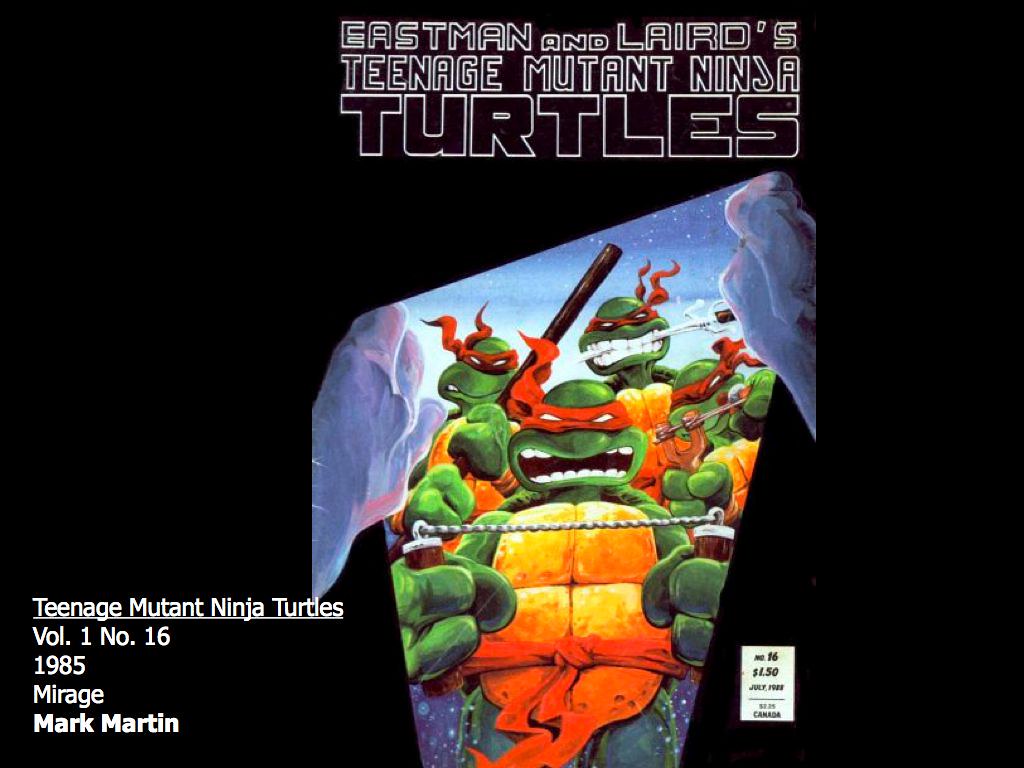The image features a single object, positioned centrally against an all-black background. This object appears to be a comic book cover from the mid-1980s, specifically the front cover of "Teenage Mutant Ninja Turtles Volume 1, Number 16," published by Mirage in 1985 and featuring artwork by Mark Martin. At the top of the cover, in black letters outlined in white, the text reads, "Eastman and Laird's Teenage Mutant Ninja Turtles." The main illustration on the cover showcases an artistic rendition of the Ninja Turtles, standing with their weapons in a snowy, partially triangular setting. The Turtles are depicted in center-bottom of the image, showcasing vibrant colors including purple, white, black, green, orange, blue, and pink. In the lower left corner of the image, the issue details are clearly stated in white font: "Teenage Mutant Ninja Turtles, Volume 1, Number 16, 1985, Mirage, Mark Martin."